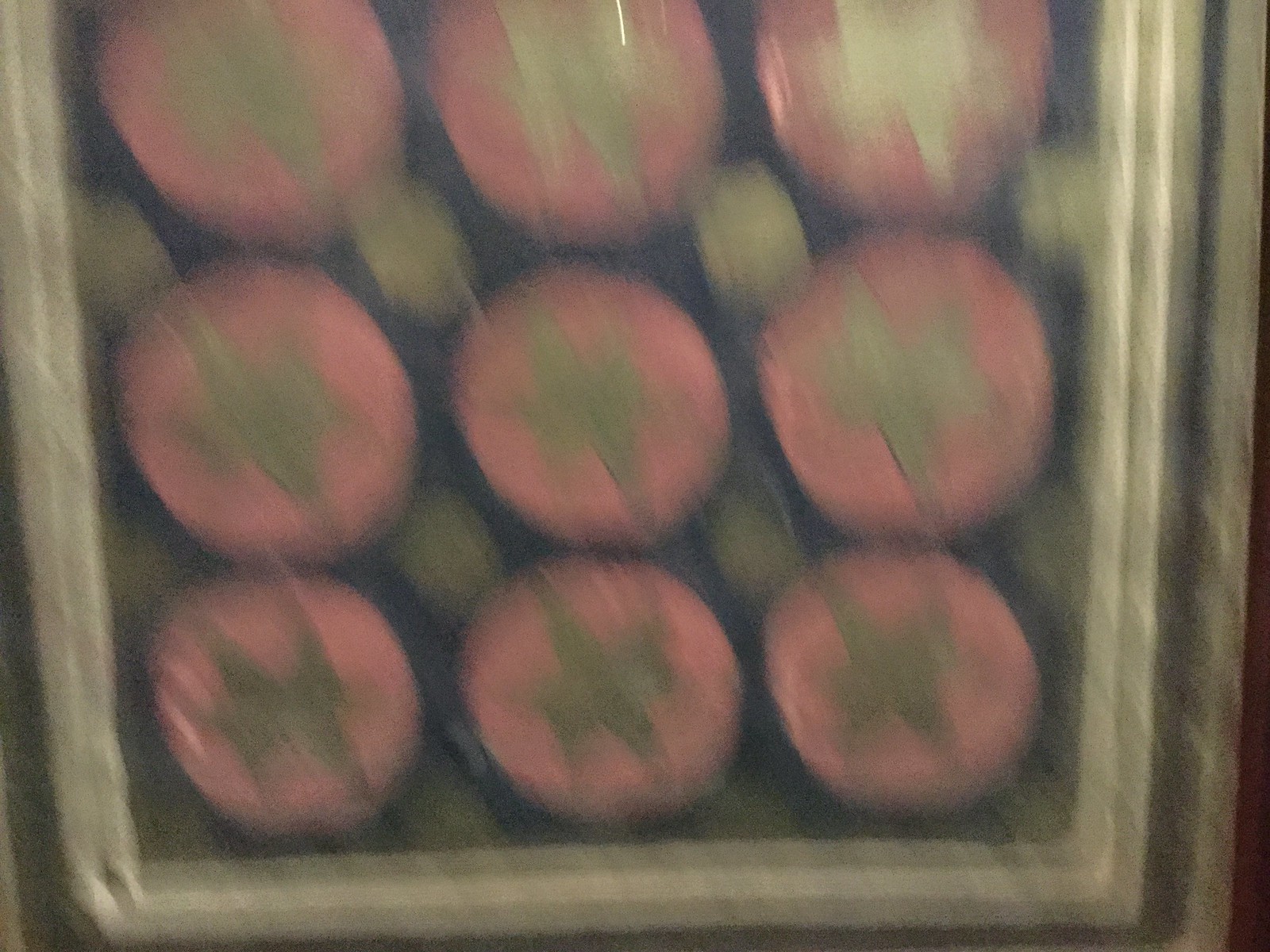In the image, an aerial view showcases a silver tray, visible on the left, right, and bottom edges. Inside the tray, three rows of muted red, circular cupcakes or cookies are organized, each circle measuring approximately 2-3 inches in height and 3 inches in width. These circles feature a drab brown, star-like shape in the center. Separating the rows are short, tan, log-like pieces resembling corks. The entire scene is set against a darker metal frame that borders the silver tray, and the image itself is quite blurry, making fine details difficult to discern.